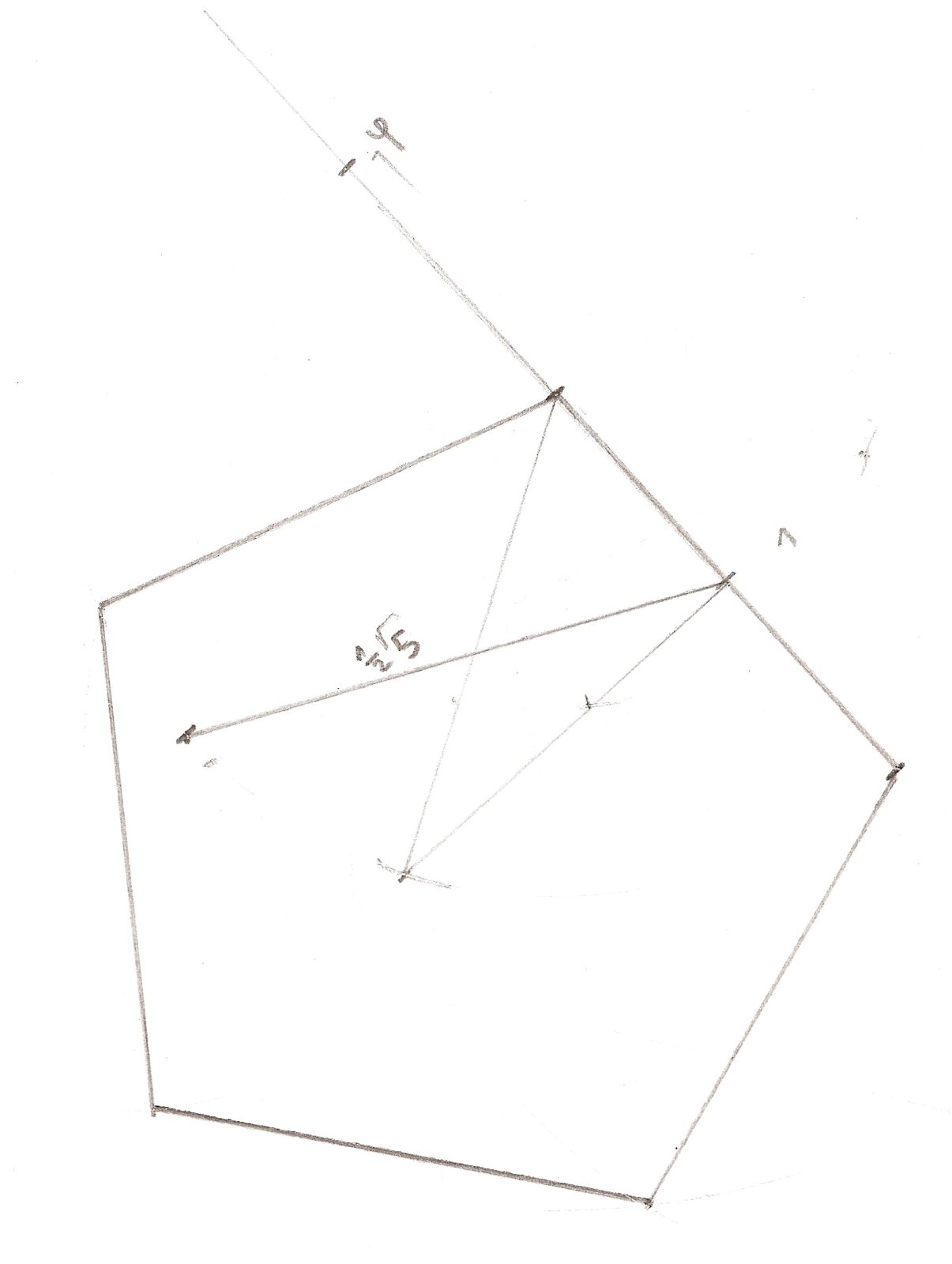The image showcases a meticulously drawn pentagon, rendered in pencil with precision that suggests the use of a ruler for the perfectly straight edges. Each of the pentagon’s five sides is uniform and exact. Inside the pentagon, two lines intersect, and one of them is labeled with what appears to be the numbers "2" and "5." Above the pentagon, the number "7" is clearly visible, and in the upper left corner of the picture, another "7" appears alongside what looks like either a letter 'Y' or a small letter 'P'. The overall attention to detail in the drawing indicates careful planning and execution.